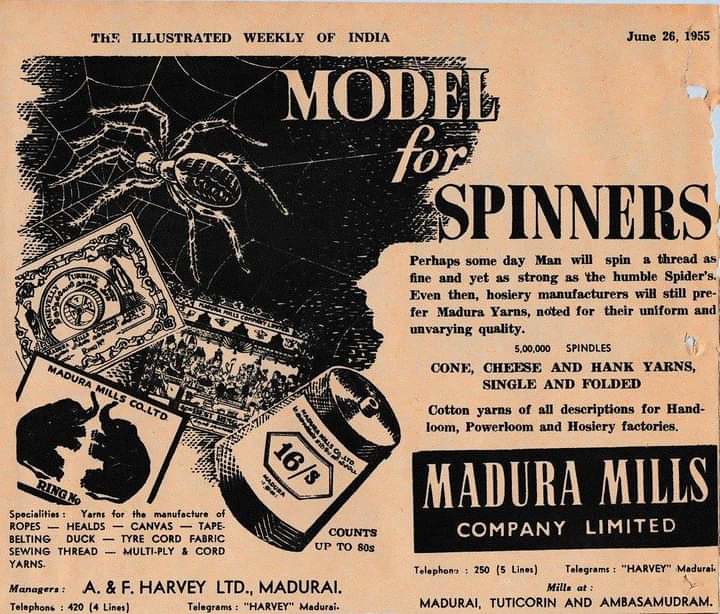The image is a yellowed and slightly torn screenshot of an advertisement from the June 26, 1955, issue of The Illustrated Weekly of India. This vintage publication features an intriguing mix of visuals and text. Dominating the left side, there is a detailed illustration of a spider on a web, reminiscent of a tarantula. Below this, the logo of Madura Mills Co. Ltd. is visible, flanked by two elephants and other smaller, less discernible logos. The centerpiece of the ad showcases a spool of thread, alluding to the product being advertised. The text, predominantly black except for the title "Model for Spinners," vividly contrasts with the yellowed paper. The main paragraph reads: "Perhaps someday man will spin a thread as fine and yet as strong as the humble spiders. Even then, hosiery manufacturers will still prefer Madura yarns, noted for their uniform and unvarying quality." The ad emphasizes the various forms of yarn available, including spindles, cone, cheese, and hank yarns, both single and folded. This nostalgic piece serves as a testament to the enduring quality and preference for Madura yarns in the textile industry.